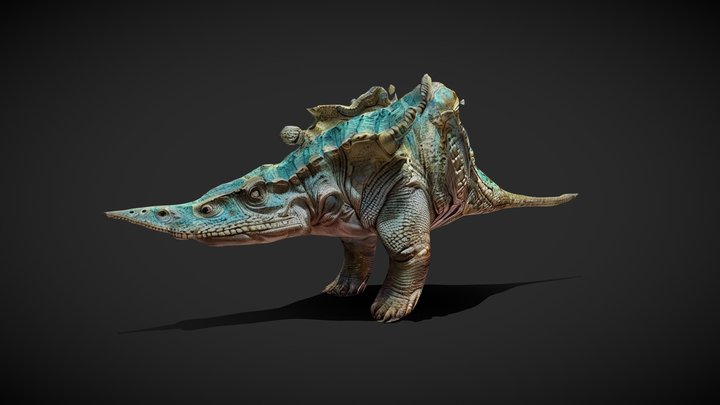The picture showcases an artistic rendition of a creature resembling a dinosaur or an iguana, set against a black or dark gray background. The subject is centrally placed in the frame, standing on two legs with a prominent and elongated snout. Its body exhibits a mixture of mint green, blue, and various shades of brown, including very light and dark brown. Distinctive features include a very long nose, a short tail, and what appears to be an armored back. The creature casts a shadow at the bottom part of the image, adding depth to the composition. The overall presentation is computer-generated, emphasizing the detailed coloration and the unique posture of the figure against the stark, textless background.